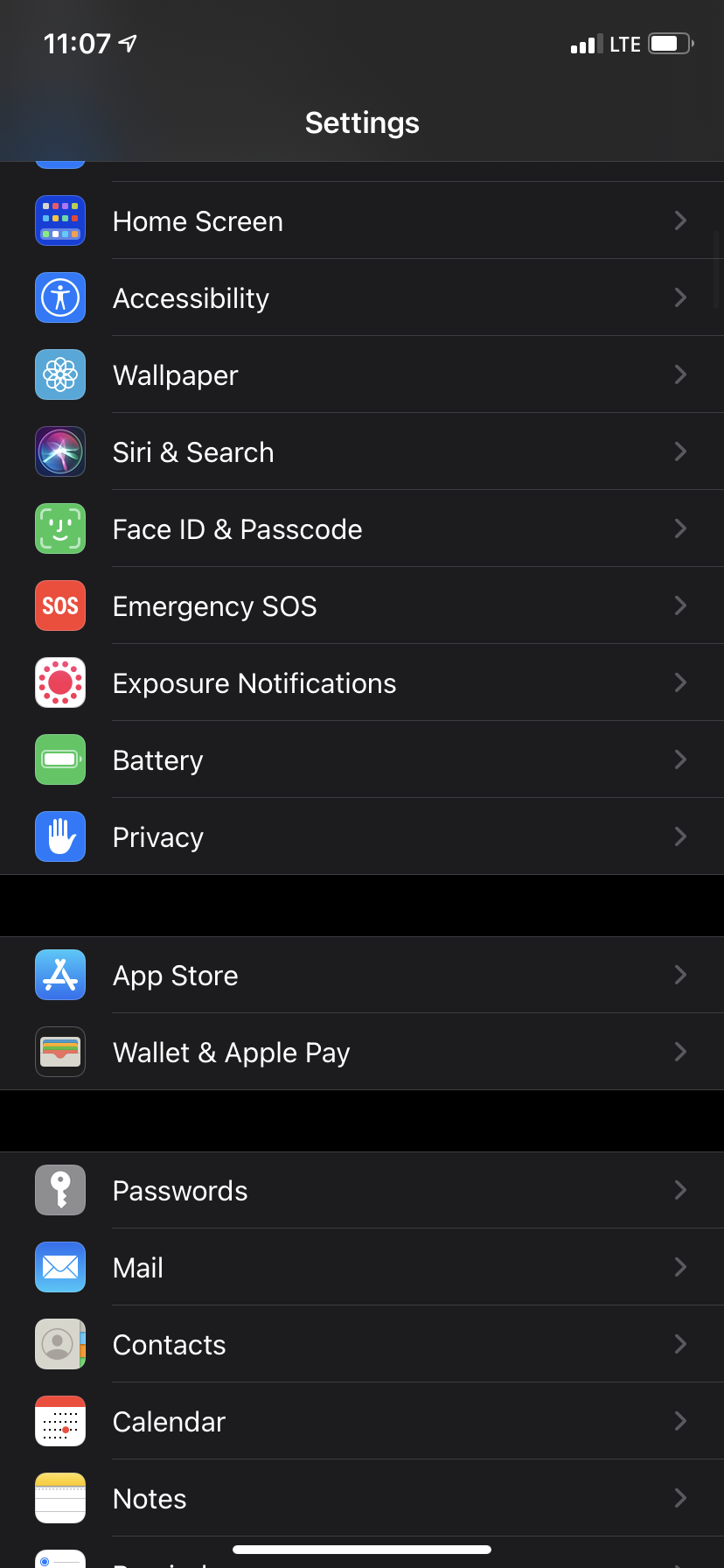This is a detailed screenshot of an iPhone settings page, captured at 11:07 AM. At the top left corner, there's an icon indicating active location services. On the top right, the status bar shows three signal bars with the network labeled "LET" in white text, a partially grayed-out signal bar, and a battery icon showing approximately 75% charge. The background of the screen is black, while the header displays "Settings" in white text.

Below the header, the settings options are listed in a light gray color with typical iPhone icons on the left and right-pointing arrows on the right, indicating further details can be accessed. The listed settings are as follows:

1. Home Screen
2. Accessibility
3. Wallpaper
4. Siri & Search
5. Face ID & Passcode
6. Emergency SOS
7. Exposure Notifications
8. Battery
9. Privacy

Following a black strip divider, the sections continue with:

10. App Store
11. Wallet & Apple Pay

Another black strip separates the next set of options:

12. Passwords
13. Mail
14. Contacts
15. Calendar
16. Notes